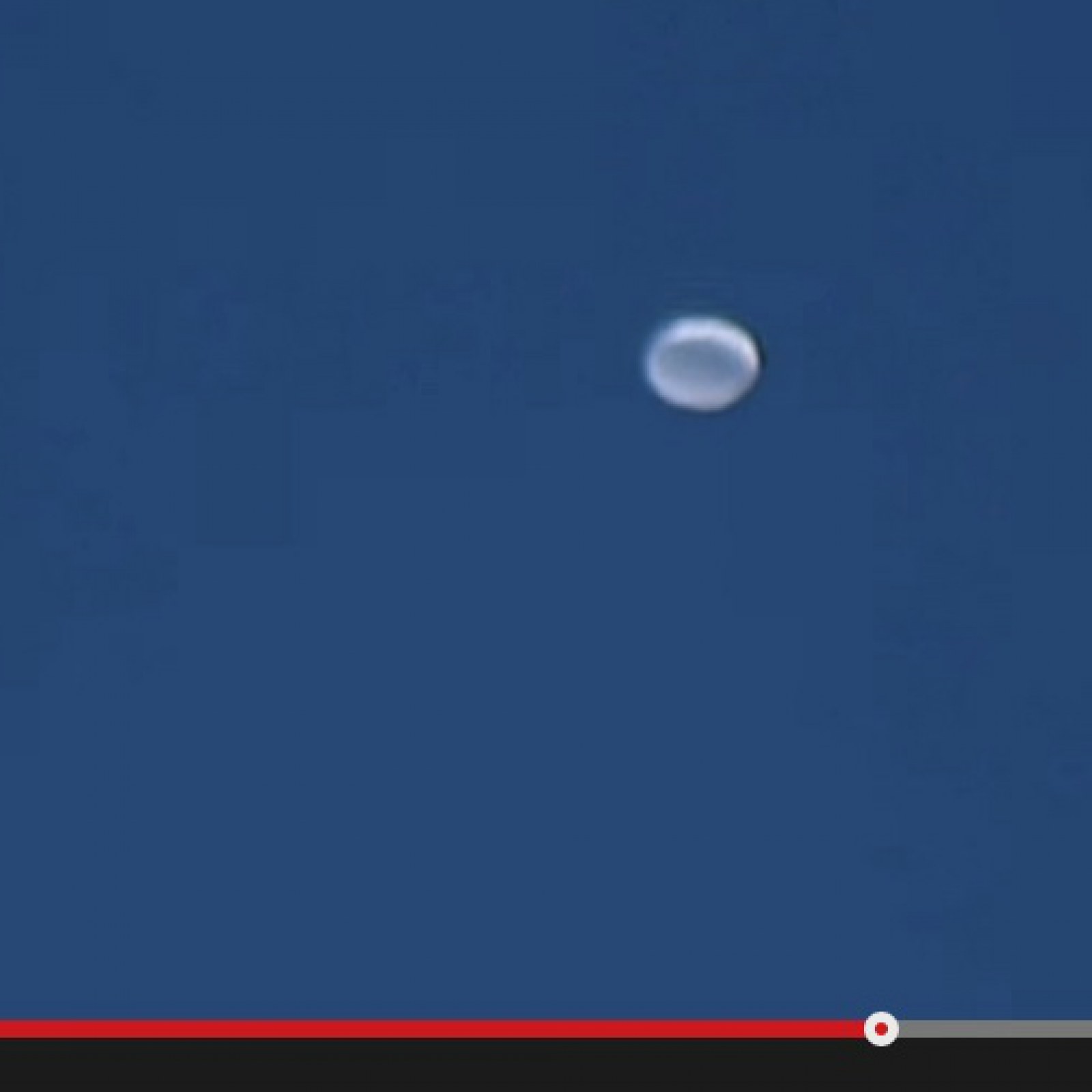The image depicts a still from a video, captured through a screenshot. The main focus is a distorted, oval-shaped white or silver sphere, which appears to be in motion or hovering in the air against a dark blue, almost grayish background. The top right of the sphere is highlighted, giving it a more luminous white appearance, while the center retains a grayish tone. The bottom portion of the image reveals the recognizable YouTube video progress bar—a red line with a white circle indicating the current play position, accompanied by gray shading representing the remaining video length. Beneath the progress bar is a black section, signature of the video's interface. The screenshot appears to be from a paused video, possibly taken for use in a presentation or to illustrate the floating sphere to someone else.